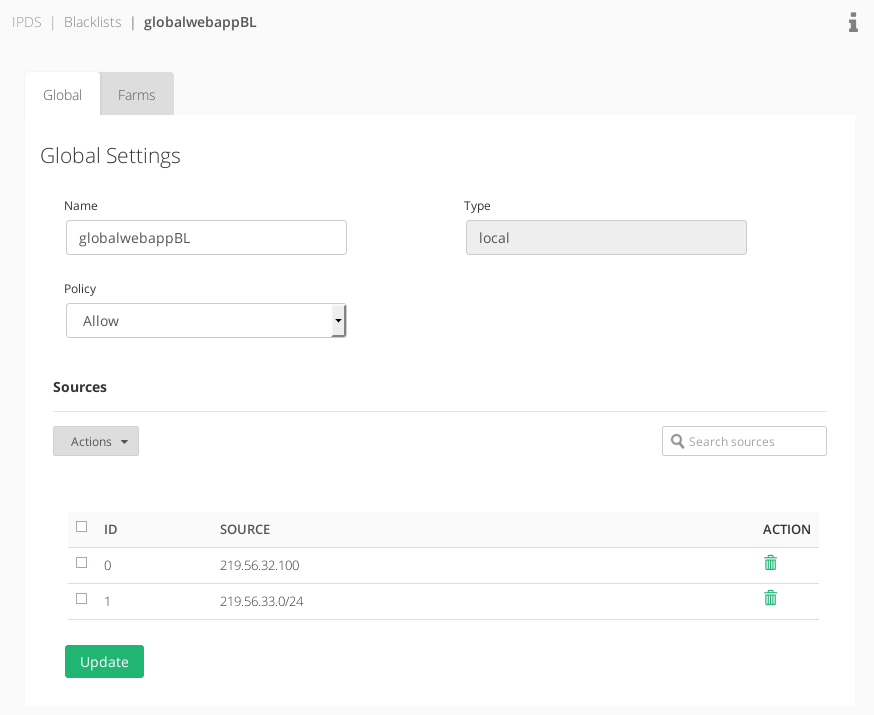In the category of websites, a specific interface section is described. In the top left corner, within a gray bar, the labels "IPDS" and "Blacklist" can be seen, followed by "Global Web App BL." To the right of these labels, there is a small information icon represented by an 'i'. Below this section, the interface features two tabs labeled "Global" and "Farms," with the "Global" tab currently active.

Under the "Global" tab, the following settings are displayed:

- **Global Settings:**
  - **Name:** Global Web App BL
  - **Type:** Local
  - **Policy:** Allow (with a drop-down menu indicating there are additional policy options, though only "Allow" is visible)

Below these settings, a section labeled "Sources" is present, which includes a drop-down menu labeled "Actions." Although other options may exist within this drop-down, "Actions" is the only visible option. Next to this drop-down, there is a search box labeled "Search Sources" accompanied by a magnifying glass icon.

The table header includes the labels "ID Source" and "Action." Below these headers, an entry is listed with the following details:
- **ID:** 0
- **Source:** 219.56.0.32, 0.100
- **Action:** Icons resembling trash cans suggest that the option to delete or retain the entry is available.